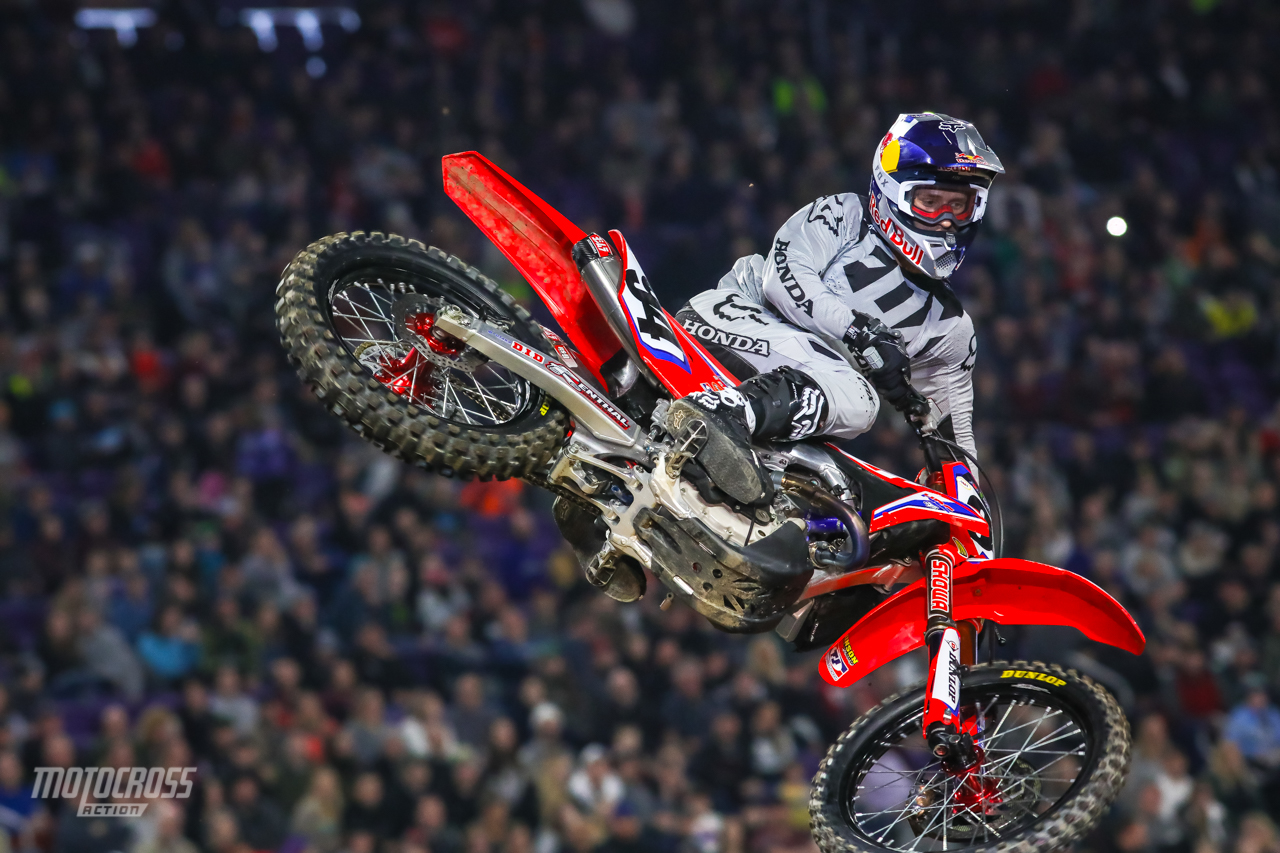The image captures a dynamic motocross rider in midair during a thrilling action shot. He is clad in a white one-piece suit adorned with various brand logos, prominently featuring "Honda" on his right leg and arm. His blue, red, and white helmet, emblazoned with the "Red Bull" logo, adds to his striking appearance. The red dirt bike he rides features the number 94 on its side and showcases black, albeit dirty, wheels that indicate a rugged use. In the backdrop, a blurred, immense crowd of spectators hints at the event's grand scale, underscoring the rider's high-flying stunt. The photograph, bearing the gray inscription "Motocross Action" in the bottom left corner, vividly portrays the adrenaline-fueled atmosphere of the motocross event.